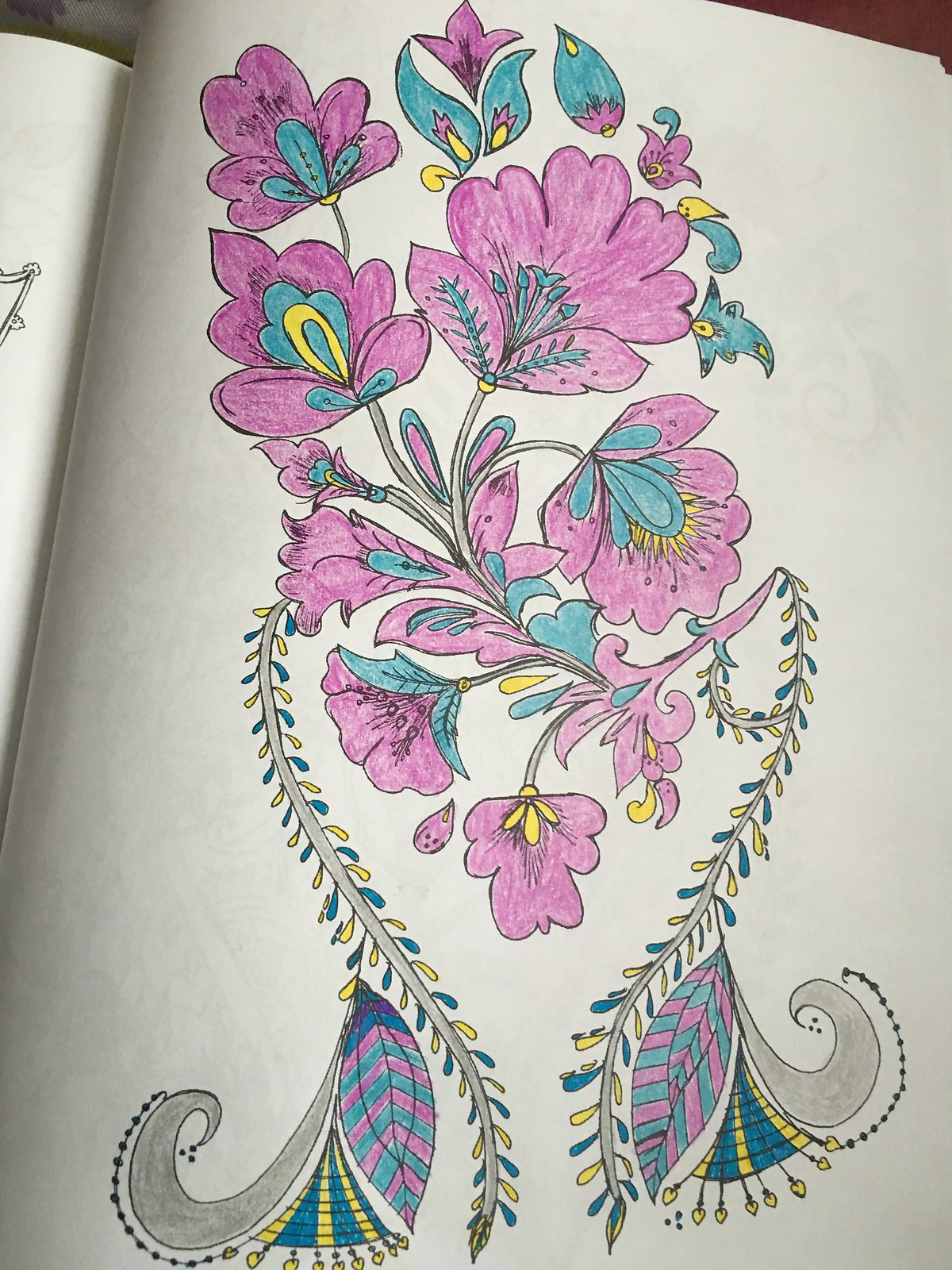The image showcases a vividly colored drawing on the plain white pages of a notebook, potentially sourced from a coloring book. Dominating the scene is a meticulously colored flower, its petals imbued with a rich shade of purple. The artist opted for a blue hue to highlight the central part of the flower, accentuating it with touches of yellow. Emerging from the blossom are a few vines, intricately colored in turquoise and yellow, adding a whimsical element to the composition. These vines gracefully extend downward before curling upwards into delicate, bell-shaped forms, consistent with the turquoise and yellow coloring interspersed with hints of gray. The artwork demonstrates a harmonious blend of colors, contributing to an overall enchanting and detailed floral illustration.